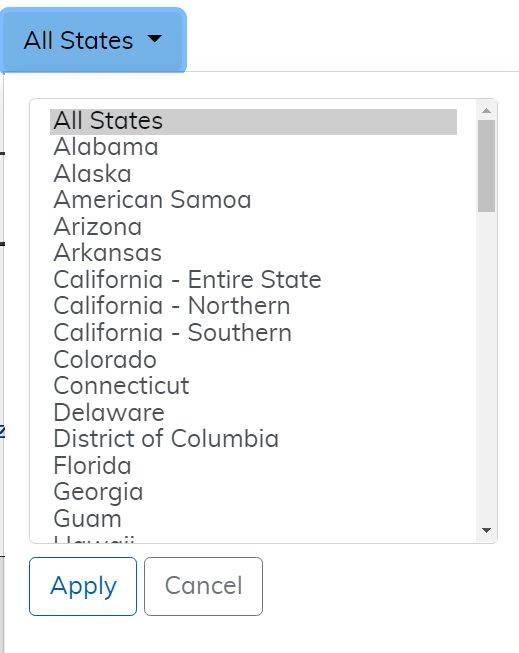This screenshot depicts a user interface for selecting U.S. states from a dropdown menu. At the top of the selection box, a thin gray line runs horizontally alongside a blue tab positioned in the top left corner. This tab is labeled "All States" in black font and is accompanied by a downward-facing arrow, indicating that it is a collapsible menu. A thin gray line also runs vertically down the left side of the box, while the right side lacks a border.

Within the dropdown menu, various state options are listed, including: Alabama, Alaska, American Samoa, Arizona, Arkansas, California (Entire State), California (Northern), California (Southern), Colorado, Connecticut, Delaware, District of Columbia, Florida, Georgia, and Guam. 

At the bottom of this interface, there are two buttons labeled "Apply" and "Cancel," allowing the user to either confirm or discard their selections. The clean layout and intuitive design ensure ease of use for selecting multiple U.S. states.